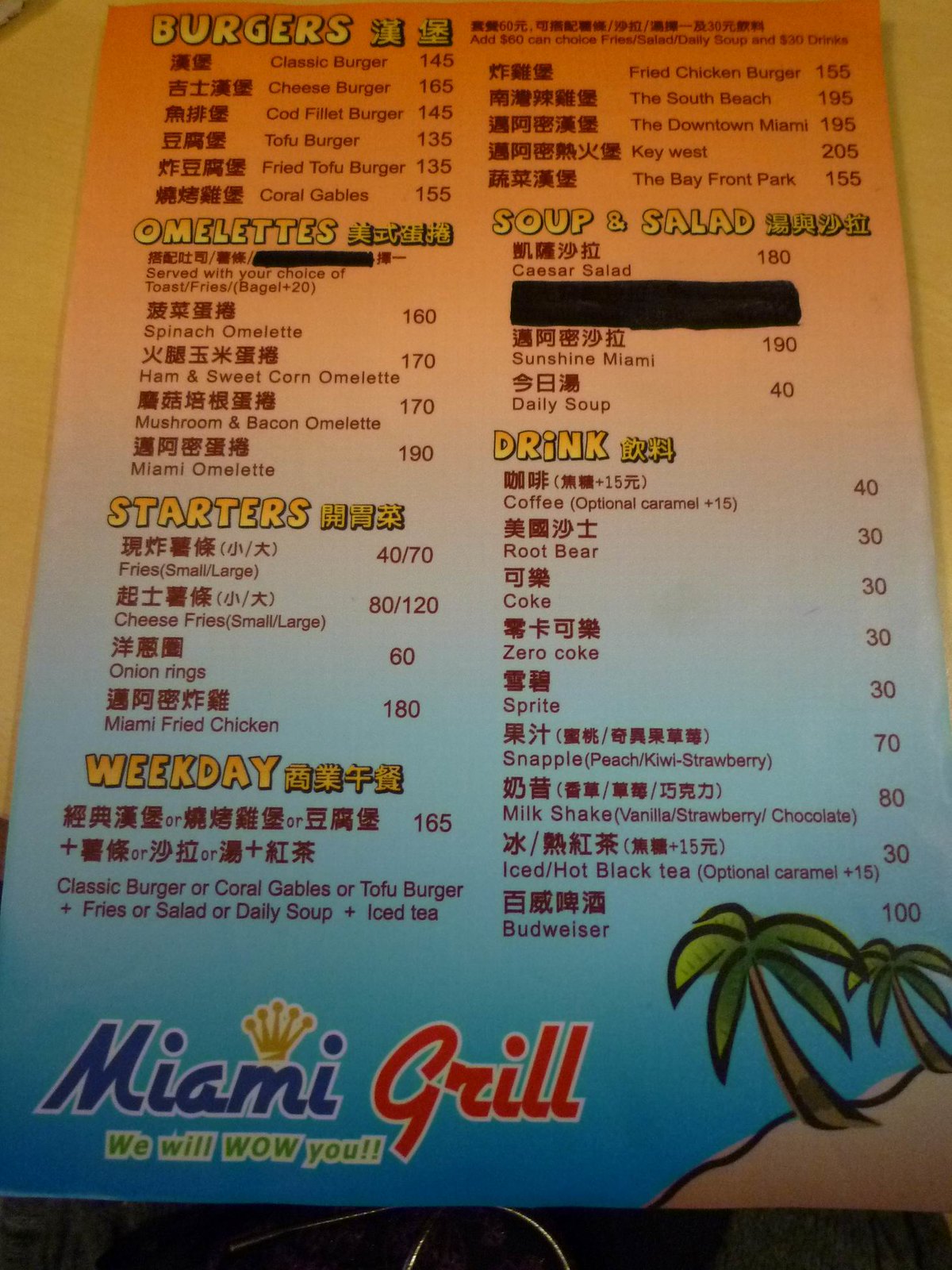Photographic image of a brightly colored menu from Miami Grill. The menu features a vibrant palette of orange, pink, and blue. Towards the right, there are cartoon-style palm trees in green and brown, rooted in a patch of sand. At the bottom of the menu, "Miami Grill" is prominently displayed with "Miami" written in a fun, blue font, and "Grill" in vivid red. A yellow crown with balls at the tips adorns the top of the 'M' in "Miami." The top of the menu boasts the slogan "We will WOW you!!" in green and white. The food items listed include various types of burgers—classic burger, cheeseburger, cod filet burger, tofu burger, fried tofu burger, and coral gables, with prices $145, $165, $135, and $155 respectively. While the currency is unspecified, Japanese or Chinese characters accompany the price listings. The menu also mentions categories like omelets, starters, weekday specials, soups, and salads. Some items appear to have been redacted with black sharpie. There's a section labeled "Drink," though it lacks further detail.